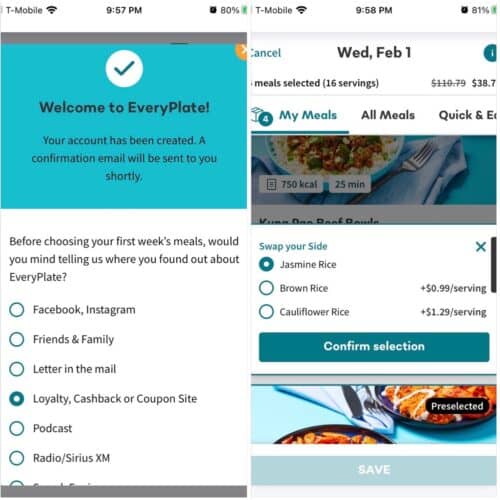The image depicts the screens of two mobile phones, displaying identical content from T-Mobile with a Wi-Fi signal and the time as 9:57 PM. The battery is at 80%, and there is an active alarm indication. 

The background of both screens is turquoise in the top left corner, with a white circle containing a turquoise check mark in the center. Below this, text reads, "Welcome to EveryPlate! Your account has been created. A confirmation email will be sent to you shortly." Further down, white text asks, "Before choosing your weekly meals, would you mind telling us where you found out about EveryPlate?" Below this question, there is a list of options, each preceded by a circle for selection. The options include: Facebook, Instagram, Friends and Family, Letter in the Mail, Loyalty Cashback or Coupon Site (with this option ticked), Podcast, Radio, and Sirius XM, among others not fully visible in the image.

On the right side of the screen, there is a 'Cancel' button aligned to the left and the date "Wednesday, February 1st" beneath it. Further down, it shows "Meals Selected: 16 servings" and a cost of "$110.79" which is crossed out, and "$38.7" displayed next to it. The bottom section of the screen has a navigation or options area with "My Meals," "All Meals," and "Quick and Easy" visible.